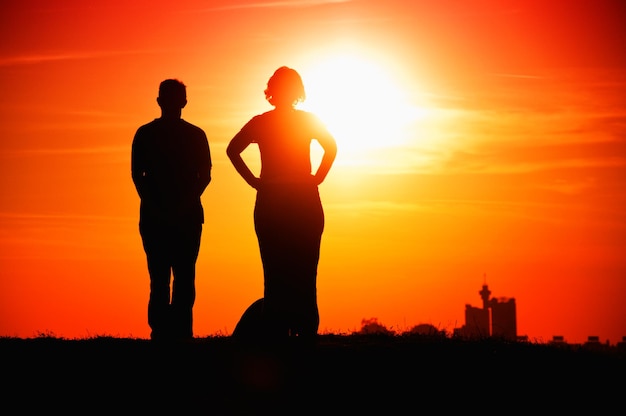The photograph captures the striking silhouette of a man and a woman standing against a breathtaking sunset. Viewed from behind, the couple faces the glowing sun, bathing the sky in harmonious hues of yellow, red, and orange. They appear to be on a hill or a flat expanse of grassy land, gazing into the amber sky. The man, distinguishable by his shorter hair and long pants, stands with his arms crossed. Beside him, the woman, identifiable by her hourglass figure and mid-length hair, has her hands confidently placed on her hips. She dons a long dress or skirt, and there seems to be a bag or backpack leaning against her leg. Behind them to the right, tall buildings and distant structures punctuate the horizon, blending into the shadowy foreground created by the sun's powerful backlight.